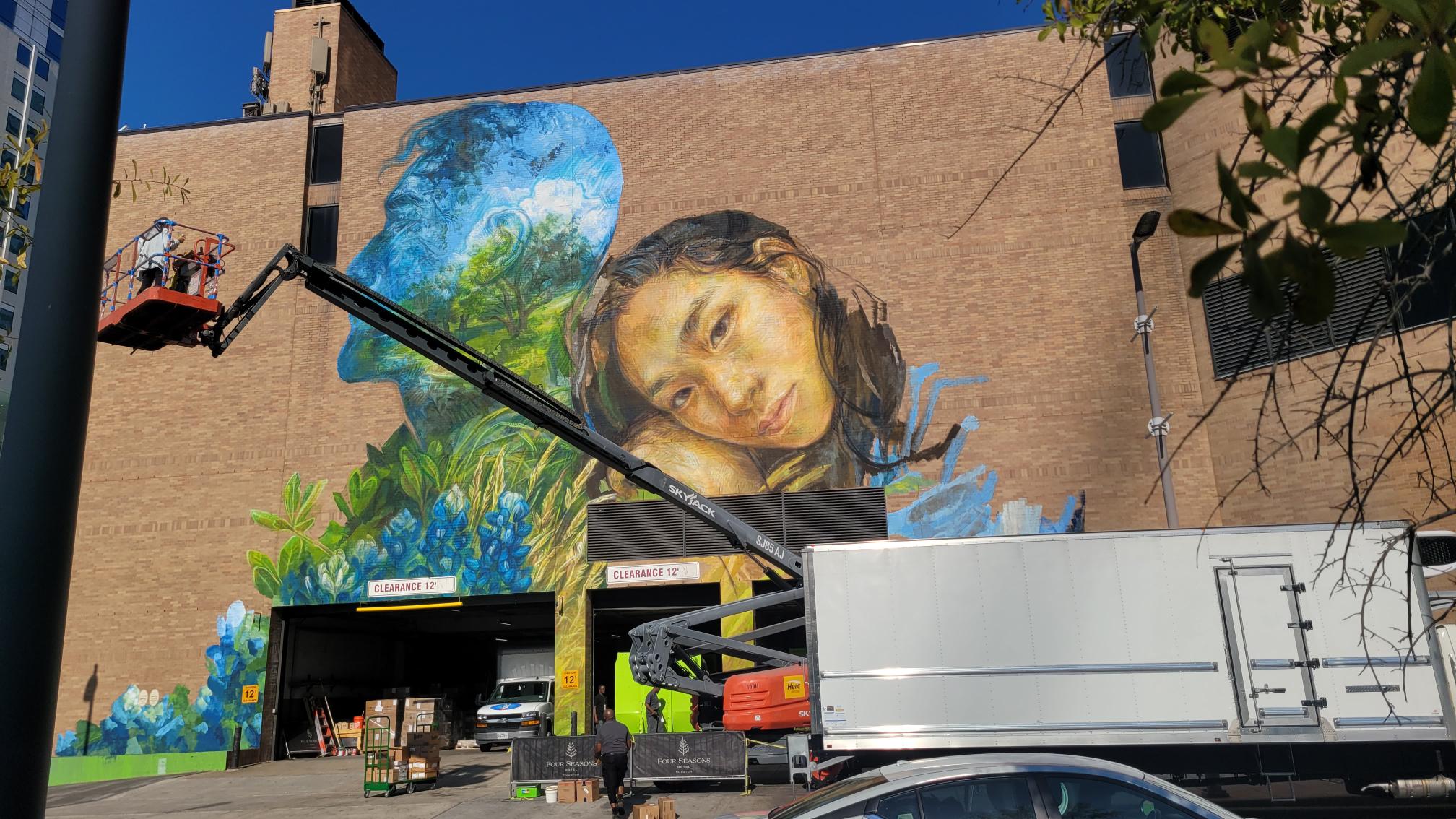The photograph captures a wide-angled view of a grand mural adorning the side of a large, square red brick building. This mural depicts a girl with long brown hair resting her head on the back of a man's silhouette. The man, facing left, is visually composed of elements from nature—blue skies, green trees, and bluebonnets—with his shoulders depicted as lush grass. Below the mural, an open garage bay reveals an ambulance inside. In the foreground, a large white moving truck is stationed at the bottom left corner, while to the right, an industrial crane with a red lift platform is visible, hoisting two people, presumably the artists, who appear to be wearing hard hats. The mural beautifully blends the human figure with natural elements, creating an evocative scene where the girl leans on a representation of nature itself.